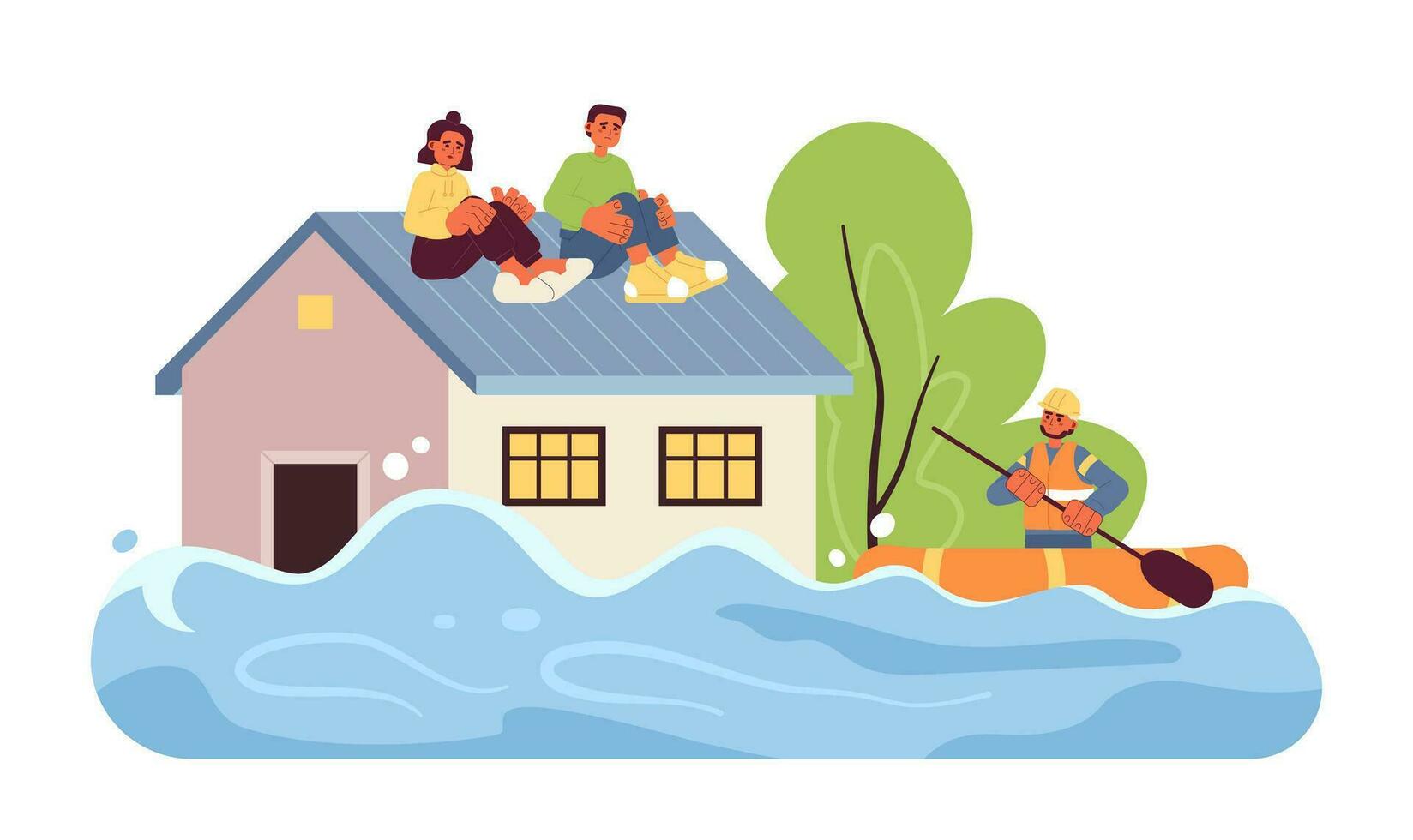In this detailed cartoon-style 3D graphic, a man and a woman are perched on the blue, triangular roof of a flooded house, seeking rescue. The house, which has a mix of pale brown and tan walls, features two prominent yellow windows with black frames, partially submerged by the rising blue waters. The roof is divided into blue planks with hints of pink on the left side. The man, positioned on the right, is wearing a green shirt, blue pants, and exaggerated yellow shoes, while the woman to the left wears a yellow shirt, brown pants, and white shoes. They sit close together, hugging their knees, against a white background.

To the right of the scene, a rescuer in an orange lifejacket, blue long-sleeve shirt, and yellow hard hat approaches them in an orange and yellow raft, paddling through the choppy water. The vibrant blue water cascades against the house, emphasizing the flooding situation. Next to the house, to the right, stands a tree, adding to the composition’s depth. The contrast between the urgency of their predicament and the stylized, exaggerated features of the characters—including their large shoes and hands, and small heads—adds a unique touch to this evocative scene.